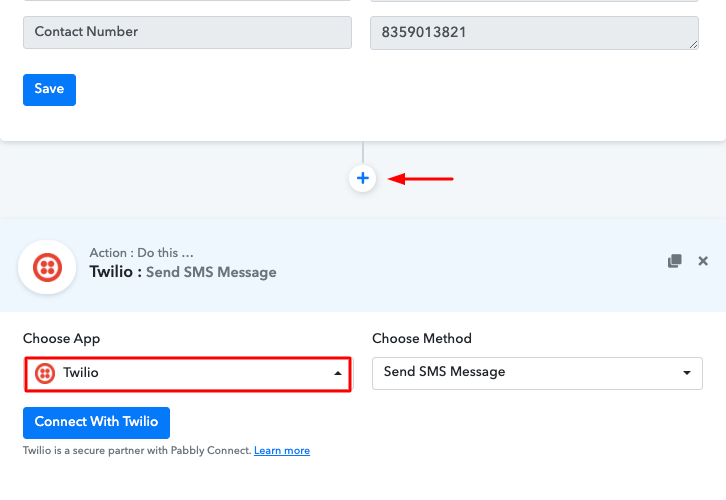The image appears to be a screenshot from an app's user interface that is focused on setting up an SMS-based action using the Twilio service. 

In the upper left-hand corner, there's a gray box with the black text "Contact Number." Directly to the right of this box, another gray box is displayed containing the contact number "8359013821" in black text.

Below the "Contact Number" label, there's a blue clickable box labeled "Save" in white text. Just beneath this, a white circle contains a prominent blue plus sign, with a red arrow pointing towards it from the right.

Further down, there's a light blue box featuring an icon of a circle with four dots inside. To the right of this icon, the text reads "Action, do this." Below this, the text "Twilio" followed by "send SMS message" is displayed. To the right, an icon resembling a dialogue box and another icon that appears to be an Xbox logo are present.

Underneath, the text "Choose app" is written in black, followed to the right by "Choose method." Directly below "Choose app," a red highlighted box with a red circle and four red dots (similar to the previous icon) reads "Twilio." Below "Choose method," another box displays the text "Send SMS message."

At the bottom of the interface, a blue, clickable box with white text states "Connect with Twilio." Underneath this, the description "Twilio is a secure partner with Pably" is noted. Additionally, the phrase "Learn more" is also clickable.